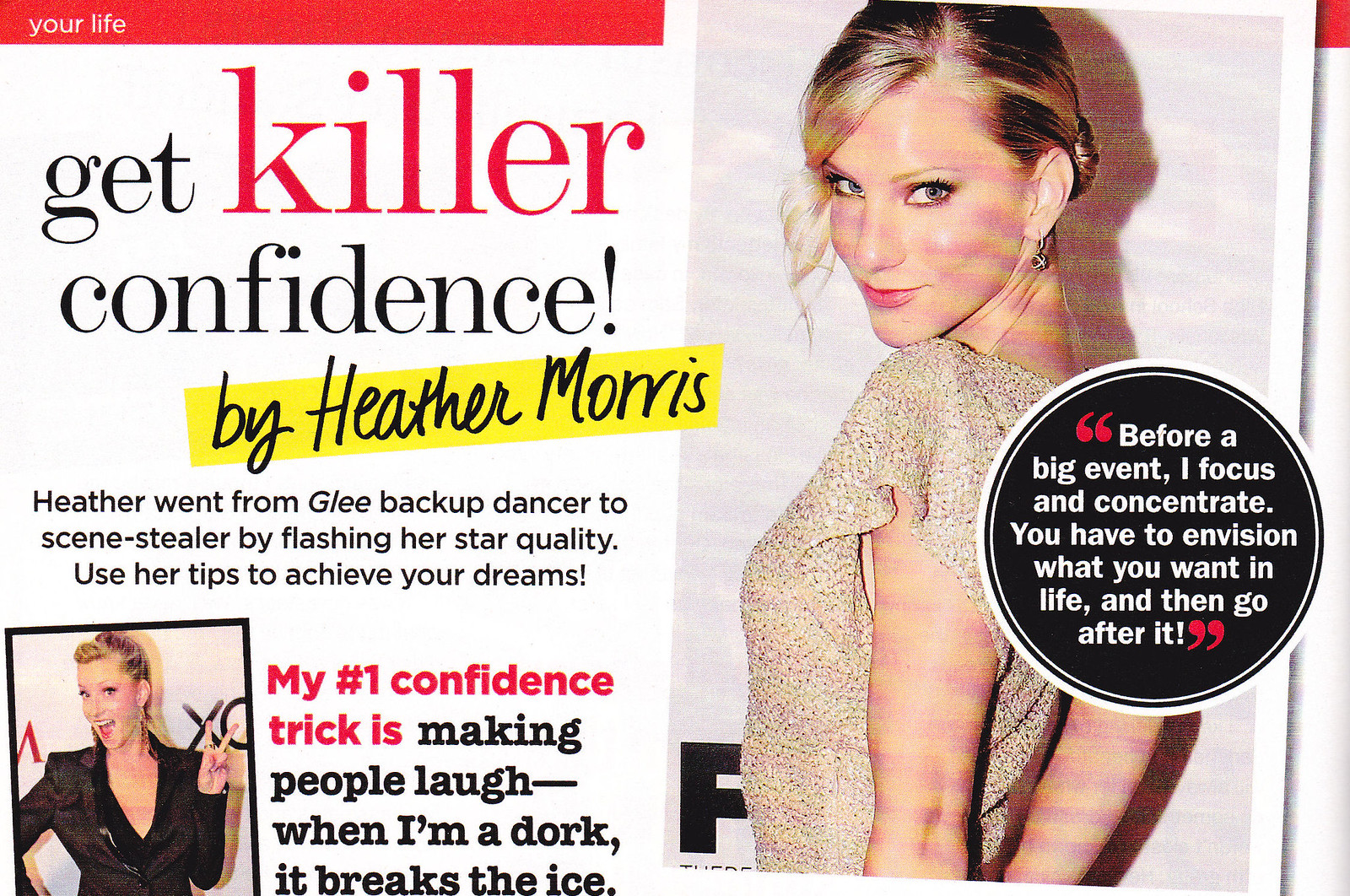This image features an inner magazine page from "Your Life" with a vibrant layout. Dominating the upper left, a prominent red bar with white text proclaims, "Your Life," followed by a bold black and red headline, "Get Killer Confidence." Below, on a yellow background, black text attributes this piece to Heather Morris. The subtitle highlights Heather's journey from a backup dancer on "Glee" to a scene-stealing star, emphasizing her star quality. It encourages readers to follow her tips to achieve their dreams.

In the lower left, there's a candid photo of Heather giving a peace sign, accompanied by her quote: "My number one confidence trick is making people laugh. When I'm a dork, it breaks the ice." On the right, Heather is elegantly posed in a gold party dress with her hair pulled up, a stylish swirl near her right ear, and earrings. She's looking down her left shoulder towards the viewer. A circular text spotlight next to this image reads, "Before a big event, I focus and concentrate. You have to envision what you want in life and then go after it." This detailed layout and empowering narrative capture Heather Morris's journey and confidence tips vividly.